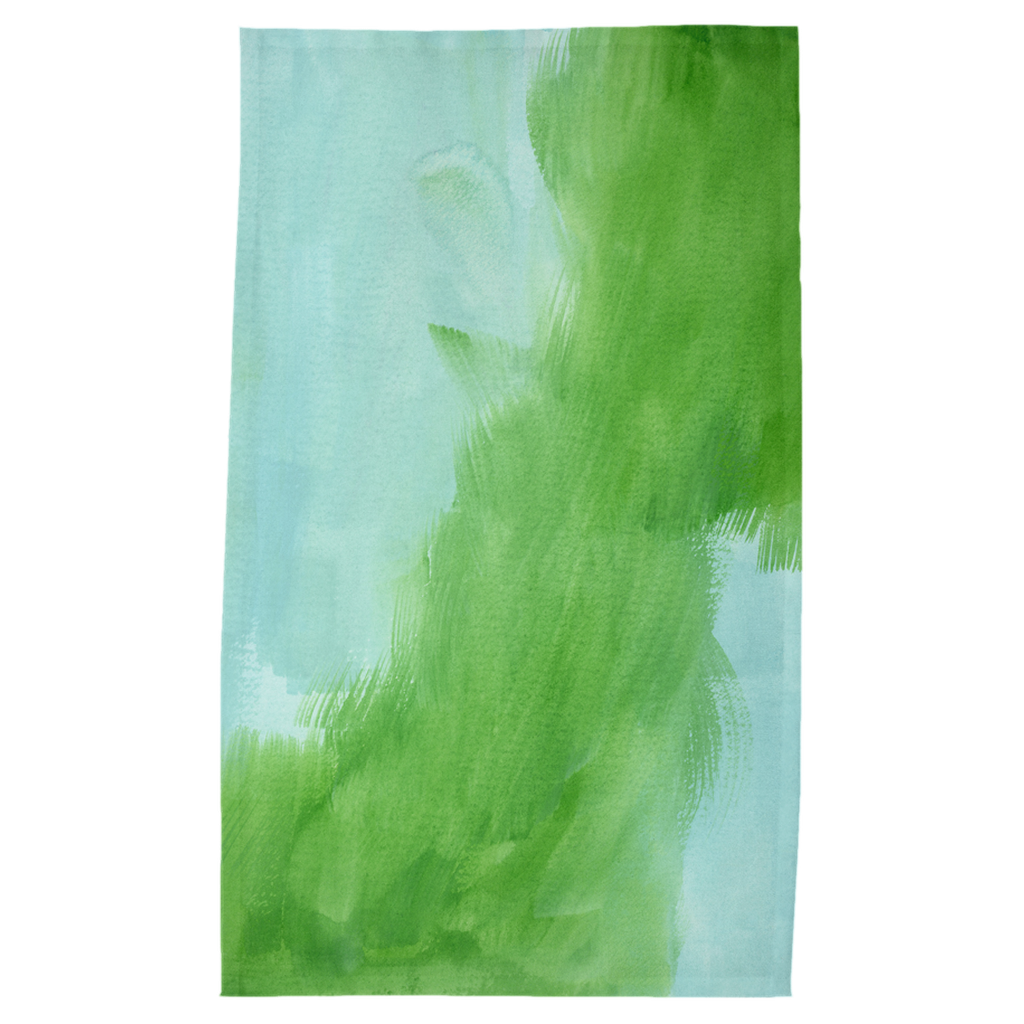This image showcases an abstract painting, likely created using watercolors, depicts a dynamic interplay of green and blue hues. The background is primarily light blue with streaks of lighter blue, creating a soothing sky-like effect. The foreground features prominent, irregular brush strokes of varying shades of green—dark green, grass green, and light green—forming an amorphous shape that extends from the lower left up to the top right-hand corner. This green form is characterized by its fluid, tapered strokes which compellingly draw the eye across the composition. Notably, there are patches where the blue background merges with white, providing subtle shading near the bottom left of the piece. The largest area of light blue is concentrated on the left side, adding balance to the image. This impressionistic and abstract work captures the viewer's attention with its vibrant yet harmonious color palette and expressive brushwork.